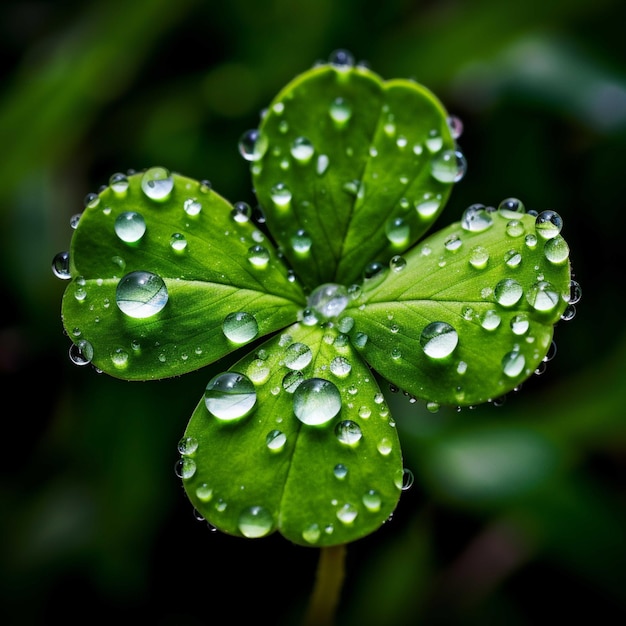This detailed macro image captures a vibrant green four-leaf clover adorned with copious dewdrops, each uniquely reflecting surrounding colors. The close-up reveals intricate veins in the leaves, enhancing the textural detail. The dew, varying in size, forms a mesmerizing spectacle of transparent beads possibly numbering around 60 to 70, displaying hues of green, purple, blue, and subtle dark shades. Set against a blurred, multi-toned green background, the clover's stem is also visible, contributing to the image's depth. The photograph exhibits signs of heavy modification, likely in Lightroom, optimizing shadows and contrast to make the clover the undeniable focal point.